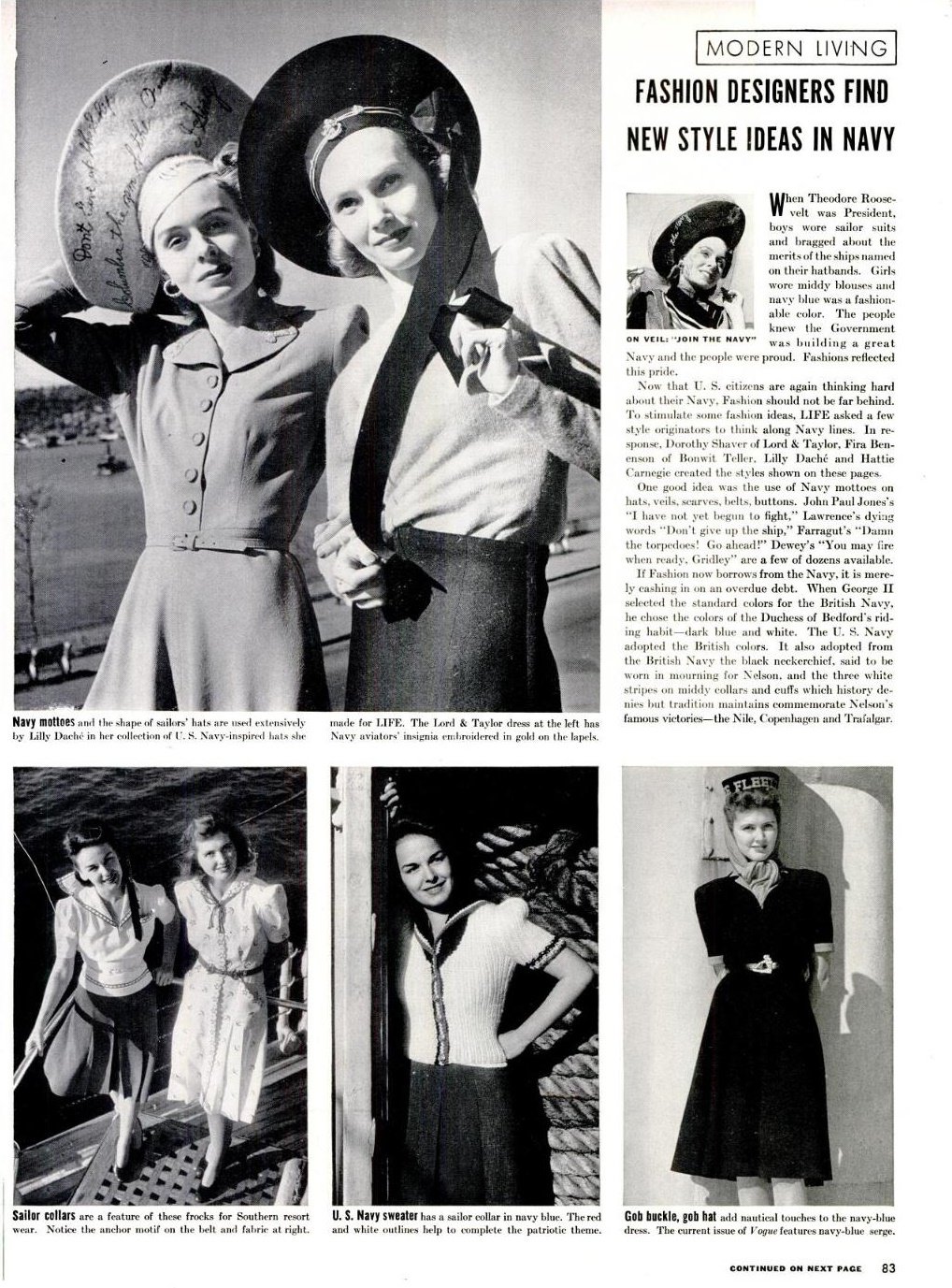The image is a black-and-white page from an old magazine, possibly from the 1950s, featuring an article titled "Modern Living: Fashion Designers Find New Style Ideas in Navy." Dominating the top left is a large photo of two women, identified as "Navy Mothers," wearing large, flat hats and dresses, their heads slightly tilted and looking ahead. To the right of this image, there's a vertical column of text and a smaller square photo of a woman in a large navy hat embedded within this text. 

The bottom half of the page is divided into three distinct images. On the far left, two women appear to be on a boat, dressed in outfits labeled "Sailor Collars" – one in a large collared white shirt paired with a pleated darker skirt, and the other in a white floral print dress. In the center, a woman is pictured in a U.S. Navy-inspired sweater, featuring short sleeves with two blue bands around the edges and a navy blue sailor collar adorned with white stripes. On the far right, another woman wears a darker black, short-sleeved dress with a flat-topped hat emblazoned with "Fleet," secured by a scarf. The overall aesthetic of the page, with its detailed fashion images and comprehensive text, captures the era's fascination with nautical influences in women's fashion.